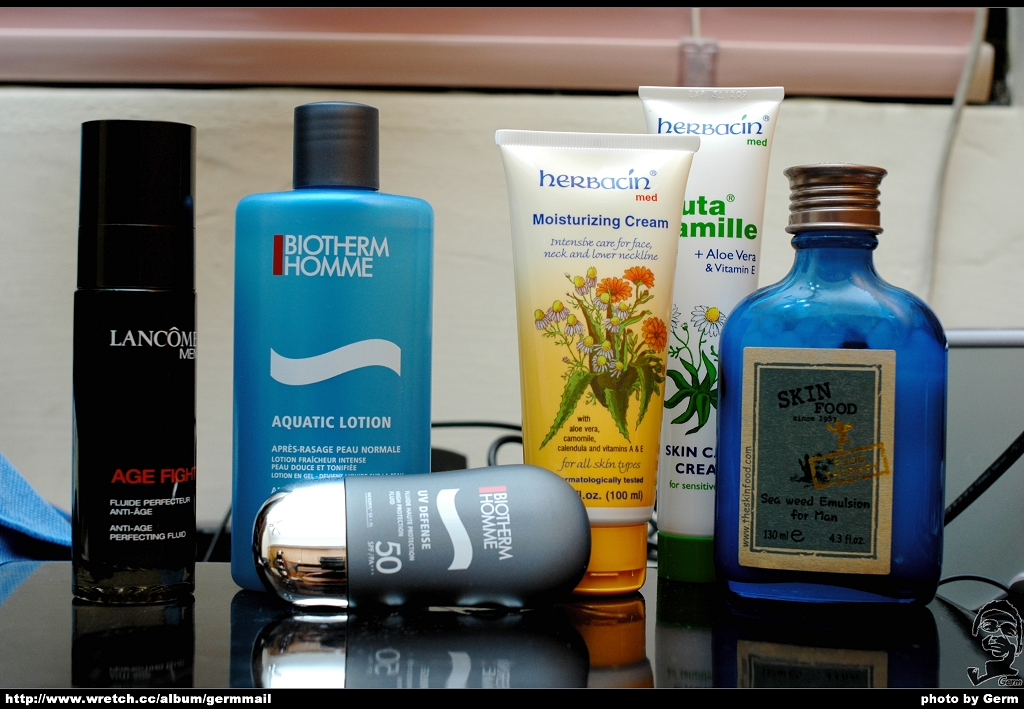On a sleek, shiny black surface, likely a nightstand or bathroom countertop, six carefully arranged skincare items are displayed against a backdrop of a white wall with visible cords. To the left, a blue cloth or rag lies next to a Lancome For Men anti-aging product. Adjacent to this, a larger blue bottle of Biotherm Homme aquatic lotion stands tall. Just below and slightly to the right, a compact gray bottle of Biotherm Homme SPF UV 50 sunscreen nestles snugly. Upright to the right of this trio is a Herbison moisturizing medical cream, followed closely by a Herbison chamomile, aloe vera, and vitamin E skincare cream. The lineup concludes with an elegant blue bottle labeled "Skin Food" on the far right.